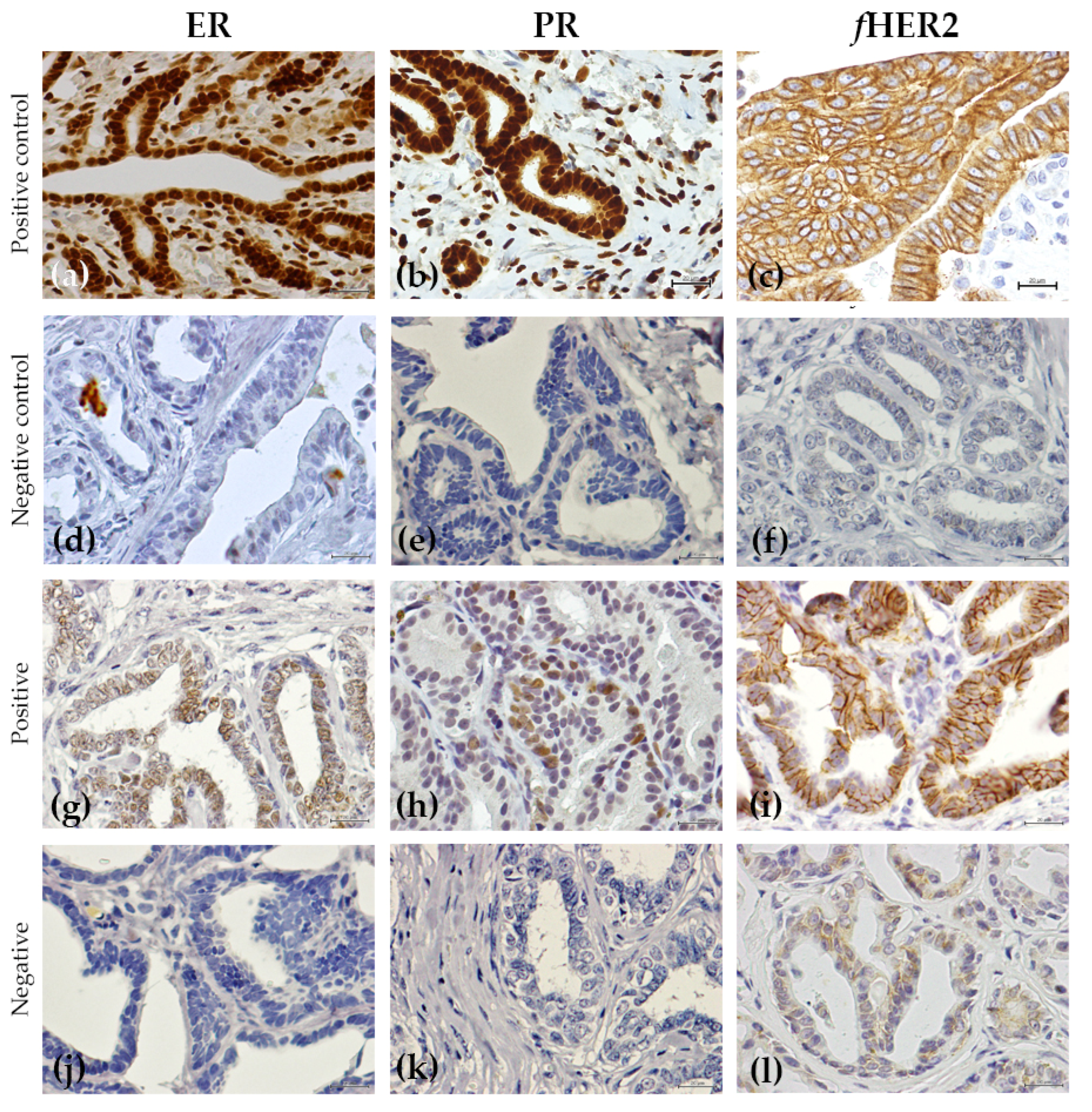This image is a detailed chart in portrait orientation, divided into three columns and four rows, reminiscent of a microscopic slide overview. Each column is labeled at the top with large black letters: ER, PR, and F HER2. Vertically, the rows are labeled on the far left as positive control, negative control, positive, and negative. The images within the chart are further divided into square segments, each labeled with letters from A to L, moving left to right, top to bottom.

The visual content of each segment consists of various cell structures or patterns that seem to resemble biological specimens under a microscope, characterized by wavy lines and circles. The color palette across these images includes shades of black, white, gray, brown, purple, blue, and off-white. Specifically, the topmost row displays more brownish hues, the second row features cells with light gray or blue tones, the third row has a mix of brown and purple shades, and the bottom row showcases predominantly bluish colors. This intricate display likely relates to the analysis of cells, potentially for medical purposes such as examining cancer cells.